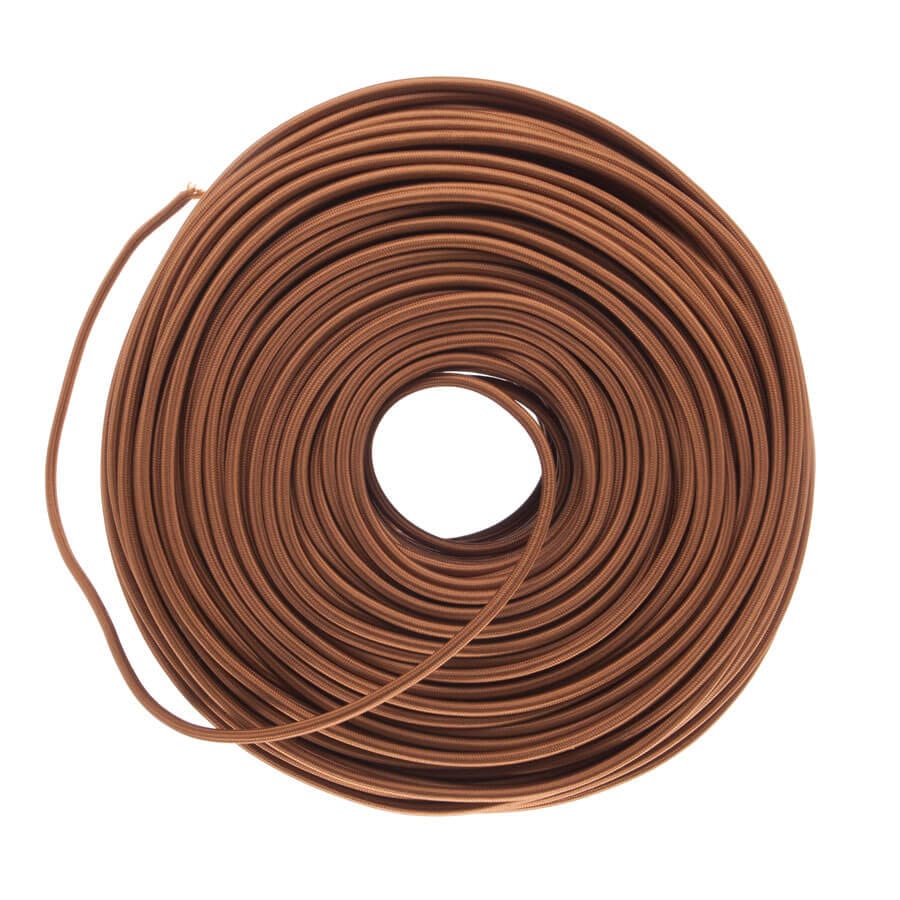This image is a highly detailed photograph of a long, thin brown string that could possibly be a braided, slightly shiny wire or leather threading. The string is bundled into a large, symmetrical circle that is centered in the frame. The dense, concentric loops give the appearance of a spool, with the string wrapping around itself dozens of times to form a thick coil. A small hole in the middle reveals a plain white background, which is consistent throughout the image. The loose end of the string emerges from this central opening, winding out towards the left side of the image and terminating with a slightly frayed tip in the upper left corner. The overall texture suggests a heavy-gauge, cylindrical thread that might be used for crafting items like moccasins or handbags.